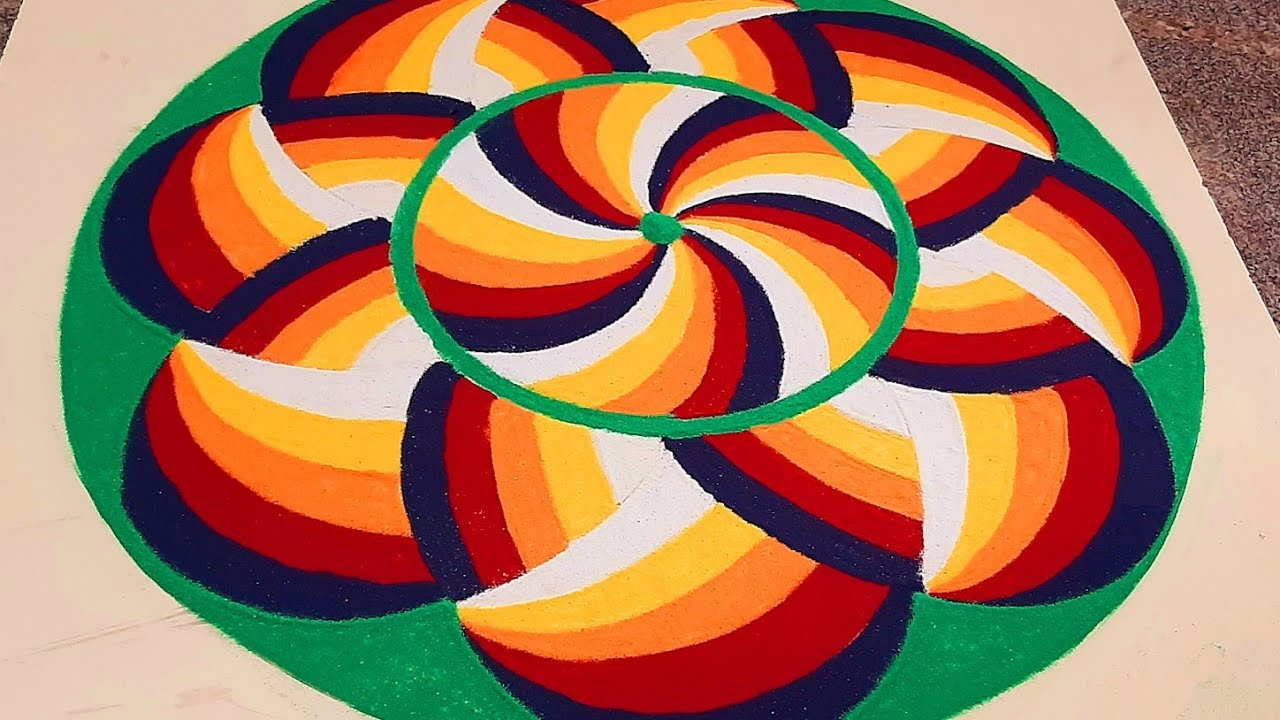This image features a geometric pattern painted on a green background. The main focus is a large circle, possibly painted on a concrete surface. This circle has a vibrant green center, around which a spiral with segments in alternating colors of dark blue, red, orange, yellow, and white curves outwards. The spiral forms multiple petals, somewhat resembling a pinwheel or flower. These patterned petals repeat beyond the central green circle, extending outward in concentric half circles, maintaining the same color scheme. The entire design is enclosed by this green circle and set against patches of what appears to be a concrete-like surface. In the upper corners of the image, there are dark brown patches, likely indicating ground or carpet. The artwork presents a harmonious yet dynamic repetition of vivid colors, making it a visually striking piece.